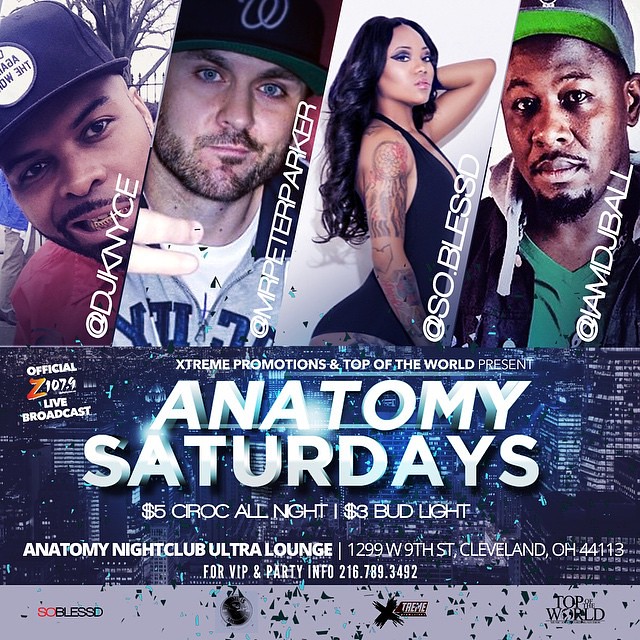This promotional poster for "Anatomy Saturdays" at Anatomy Nightclub Ultra Lounge features a vibrant and diverse collage of four individuals at the top. On the far left is DJ K-NY-C-E, an African American man sporting gold teeth, a black hat with a partially visible white circle containing the word "the," and a green-billed cap. He is followed by Mr. Peter Parker, a Caucasian man with blue eyes and a slight mustache and beard, posing with two fingers below his chin and wearing a black baseball cap with a white "W," featuring a green underside. Next is So Blessed, a woman in a black dress with tattoos along her right arm and back, facing to the right while looking towards the camera with her long black hair cascading down. The lineup concludes with I Am DJ Ball, another African American man wearing a green T-shirt, black jacket or hoodie, and a black baseball cap with a green underside that features a white logo partially obscured from view. 

Below their images, in bold white letters, is the event title "Anatomy Saturdays," with smaller text above it reading "Extreme Promotions and Top of The World present" and "Official Zed 107.4 Live Broadcast." The promotional details include "$5 Siroc All Night / $3 Bud Light" alongside the venue information: "Anatomy Nightclub Ultra Lounge, 1299 West 9th Street, Cleveland, Ohio 44113." For additional information concerning VIP and party arrangements, a contact number, 216-789-3492, is provided. The background of the poster depicts the energetic nightlife of city office towers, with various logos at the bottom including "So Blessed" on the left, another unidentified logo, "Extreme," and "Top of the World" on the far right, all set against a light gray border.